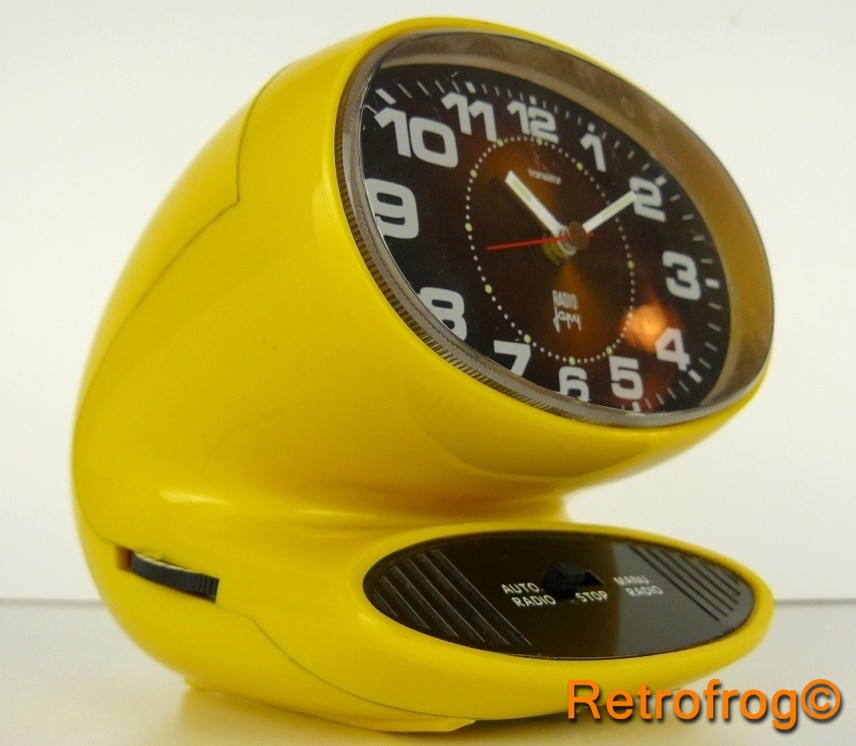The image depicts a large, retro-style, U-shaped clock device. The main body of the device is a bright banana yellow and it sits on a white or beige countertop against a white wall, slightly angled to the right. At the top center of the U-shape, there is a prominent circular clock with a black face. The clock features white numbers from 1 to 12, white hour and minute hands, and a skinny red second hand. Below the clock face, on a black oval panel, there are sections labeled "auto radio" with speaker lines on either side and various buttons, indicating that it also functions as a radio. To the left of the clock face, there is a volume control knob. In the bottom right corner of the image, the text "retro frog ©" is visible, marking it as a copyrighted image.